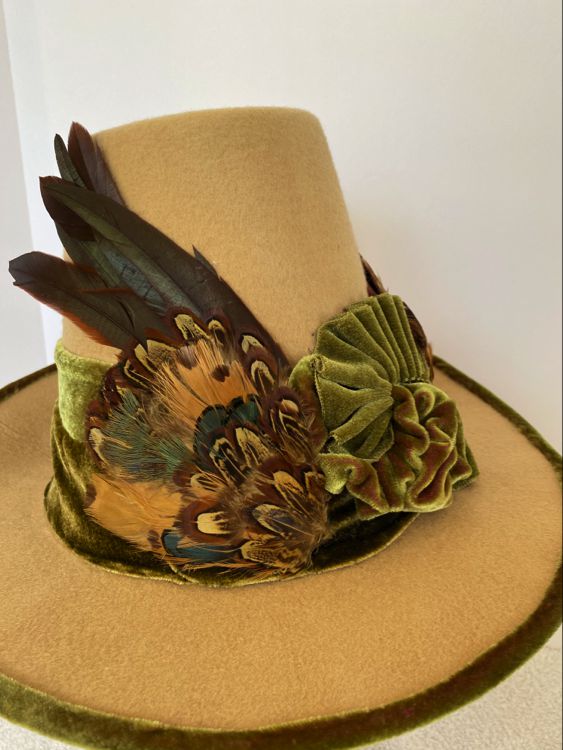This image showcases an intricately designed hat made primarily of tan, fuzzy felt material. The hat sits against a stark white background, accentuating its features. Its most striking element is the green, olive-y velvet trim that encircles the base and travels halfway up the tall crown, giving it a distinctive height. Complementing this trim is a green frilled bow positioned at the front, where the fabric overlaps elegantly.

The hat's wide brim is also adorned with the same plush green velvet, enhancing its refined appearance. A collection of vibrant feathers is tucked into the trim, adding a touch of whimsy and flair. These feathers, possibly from various birds, showcase an array of colors and patterns including black, blue, royal blue, orange, brown, and light blue. Some feathers resemble peacock plumage, contributing to the hat's eccentric and eye-catching design. The top of the hat is flat, completing its unique and detailed look.